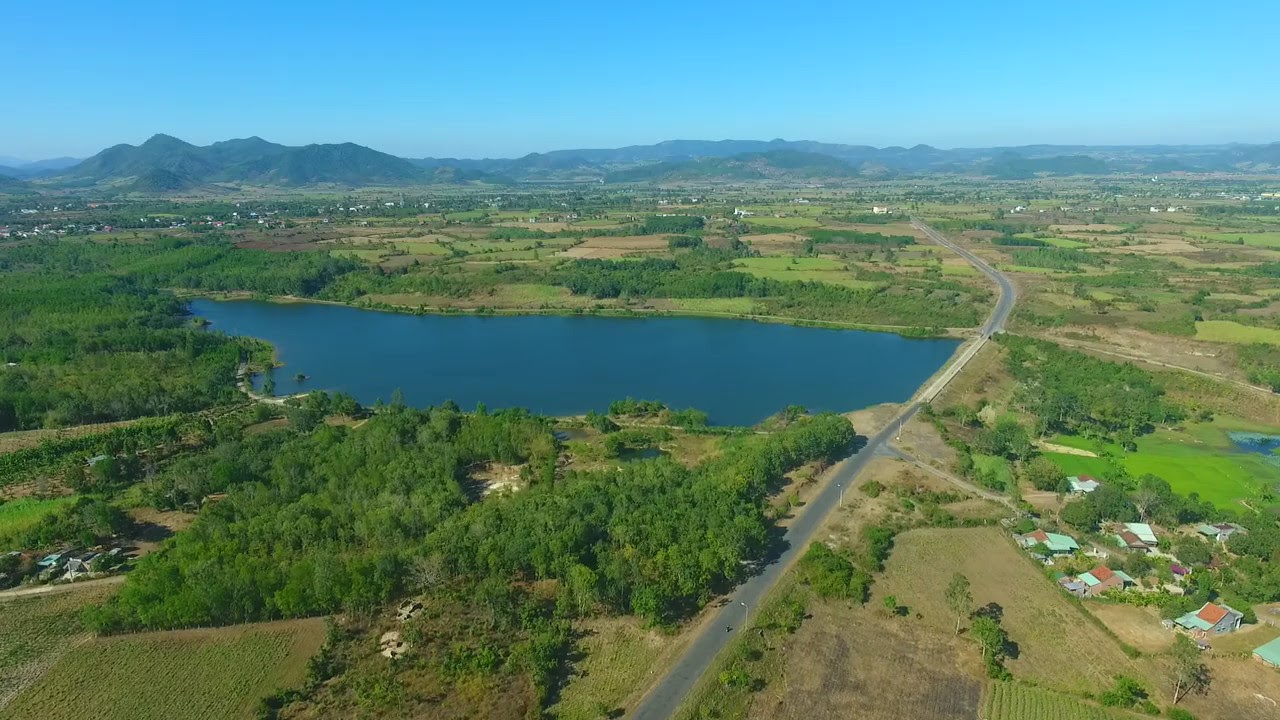This aerial photograph captures a picturesque countryside landscape, likely taken during summertime. It features a central single-lane road running vertically from the bottom of the image towards the horizon, lined with green trees and farmland. To the left of the road, approximately halfway up the image, there is a substantial body of water, appearing as a serene blue lake surrounded by lush greenery. The right side of the road showcases farmland with patches of green and fields of crops visible towards the bottom. Small communities and houses with varied rooftops—reddish, brown, and white—dot the landscape, primarily on the right side and in the distant background. The sky above is a vivid aqua color, deepening towards the top, and meets a distant tree-lined horizon that indicates a hilly terrain or mountain range. The photograph exudes a peaceful rural charm, emphasizing the abundant greenery and clear, expansive sky.